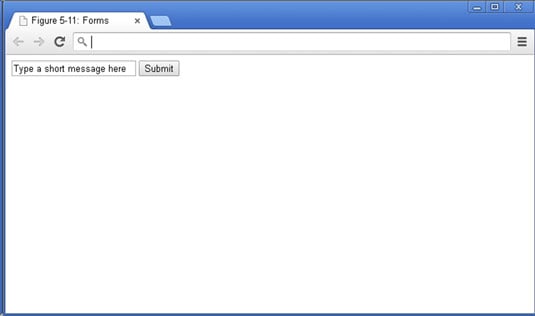The image displays a detailed web interface. At the very top, there is a medium blue banner extending to the right. On the right side of the banner, there are three small icons. The first icon is a simple white line. The second icon is a white-outlined square filled with blue, featuring a white "X" in the center. The top of the interface resembles a browser window with a tab indicated by a page icon with a folded down corner. The tab is labeled "Figure 5-11: Forms" in black print, ending with an "X."

Beneath this tab section, there are two navigational arrows pointing left and right, with the refresh button prominently displayed in a darker print. Below that, there is a search bar marked by a magnifying glass icon followed by a horizontal line. Exiting the search bar are three horizontally stacked lines, suggesting a menu.

The main body of the interface has a white background. At the top of this section, another search bar appears, bearing the placeholder text "Type a short message here," with "T" and "S" capitalized. Adjacent to this search bar, there is a submit button with the text "Submit" in black, and again, the "S" is capitalized.